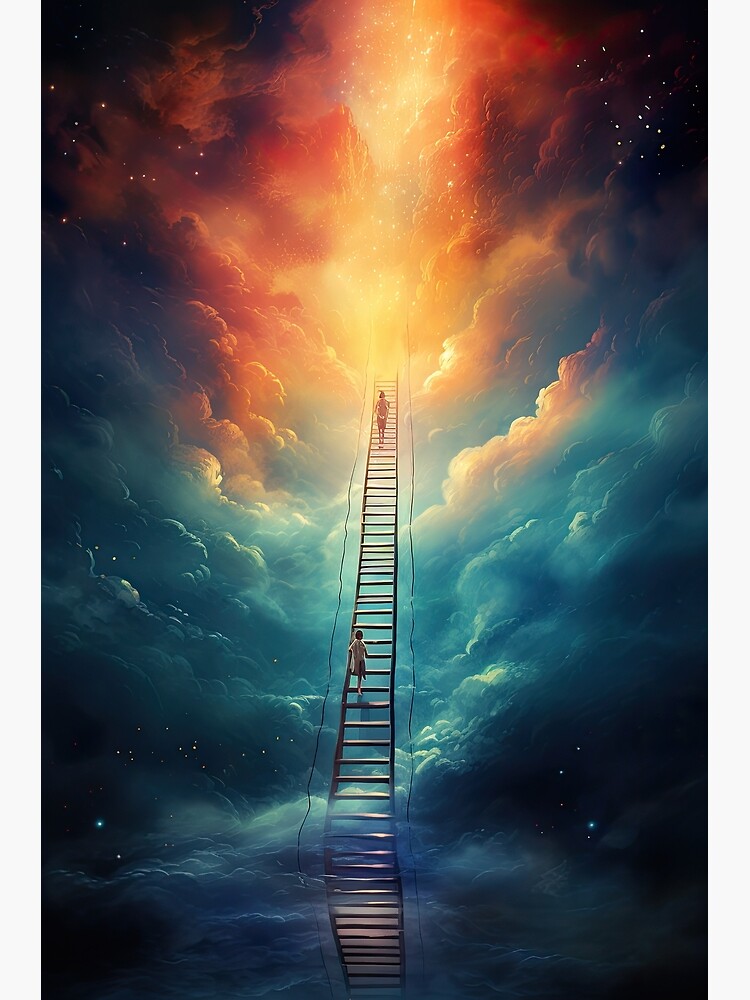This is an intricate computer-generated artwork, potentially crafted by artificial intelligence, depicting a grand staircase ascending into the clouds, reminiscent of a classical depiction of heaven. The piece is in portrait layout with steps extending vertically through the center. At the base, the scenery features dark and ominous hues of blacks, blues, and purples interspersed with white sparkles that possibly signify stars. As your eyes ascend, the artwork transitions from this eerie lower realm to a brilliant golden light at the top, where a golden shaft pierces through the clouds. This golden light gradually blends into warmer tones of oranges and reds and finally into yellowish-white at the summit, giving the impression of moving from darkness into a divine, radiant heaven.

Two indistinct figures climb the staircase, one higher up and the other lower down, their backs to the viewer, making it impossible to discern their gender, age, or race. These figures, small compared to the massive stairway, add a sense of scale and human journey to the celestial path. Around the steps, clouds with shades of blue, white, and light blue form, enhancing the ethereal and otherworldly atmosphere. The bottom of the image reflects the staircase, adding depth and symmetry to the artwork.